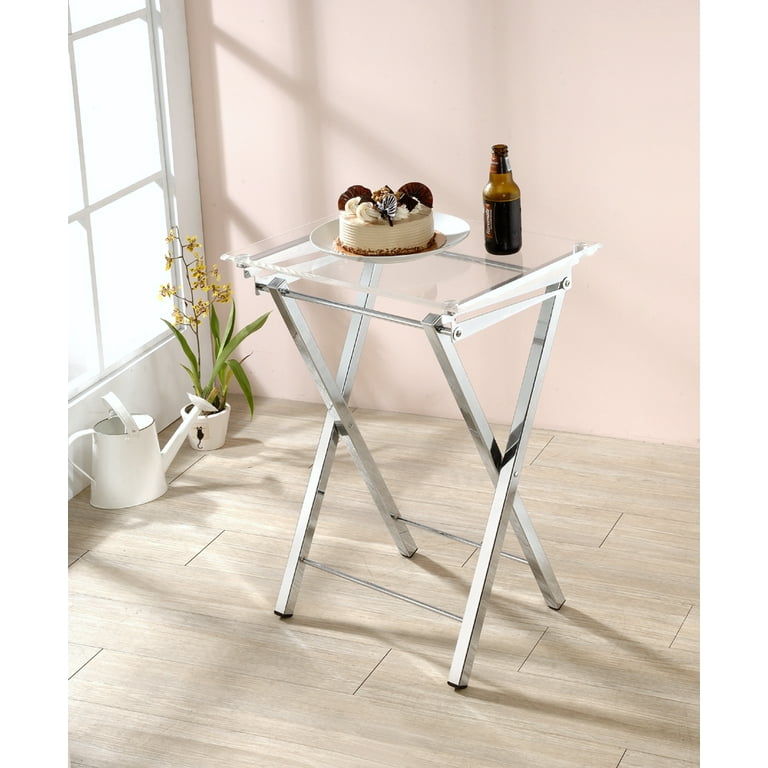In the serene ambiance of a modern apartment, a delightful scene unfolds. At the center, a minimalist TV tray with white cross legs and a glass top stands gracefully on light beech wood laminate flooring. The room basks in the golden sunlight streaming through a door situated in the upper right corner, casting a warm glow across the space. By the door, a charming white watering can sits beside a plant in a white pot. The plant boasts a tall, sturdy stalk adorned with yellow and brown petals, topped with a whimsical little black hat. Atop the stylish TV tray, a celebration awaits: a frosty beer and a beautifully crafted birthday cake. The cake, adorned in white, features elegant white swirls, two chocolate fans, and a drizzle of white chocolate on a decadent piece of dark chocolate. Each element of this happy little picture comes together to create a visually pleasing and joyous setting.